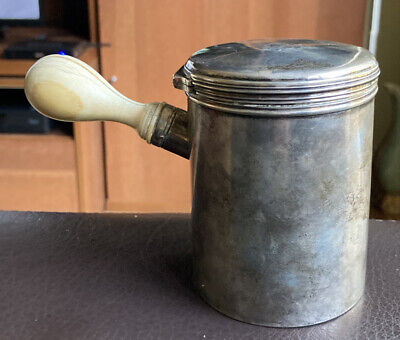The image depicts an old-time, tall, cylindrical metal canister with a screw-on lid, resembling a large cookie or flour container. The canister is silver in color and features a metal post or arm extending from its side, ending in a wooden handle that's smooth and bulbous at the end. Attached at the back is a white or cream-colored bulb with a small dark brown spot. The canister is positioned on a gray countertop or tabletop, possibly within a domestic setting. In the slightly out-of-focus background, there is an entertainment stand made of wood with visible paneling and cabinets. Partially visible are a TV screen, a DVD player, and possibly a modem box. Additionally, to the right side of the image, there's the edge of a vase. The area behind the canister also shows what seems to be a blackish-gray leather armrest of a couch or sofa.